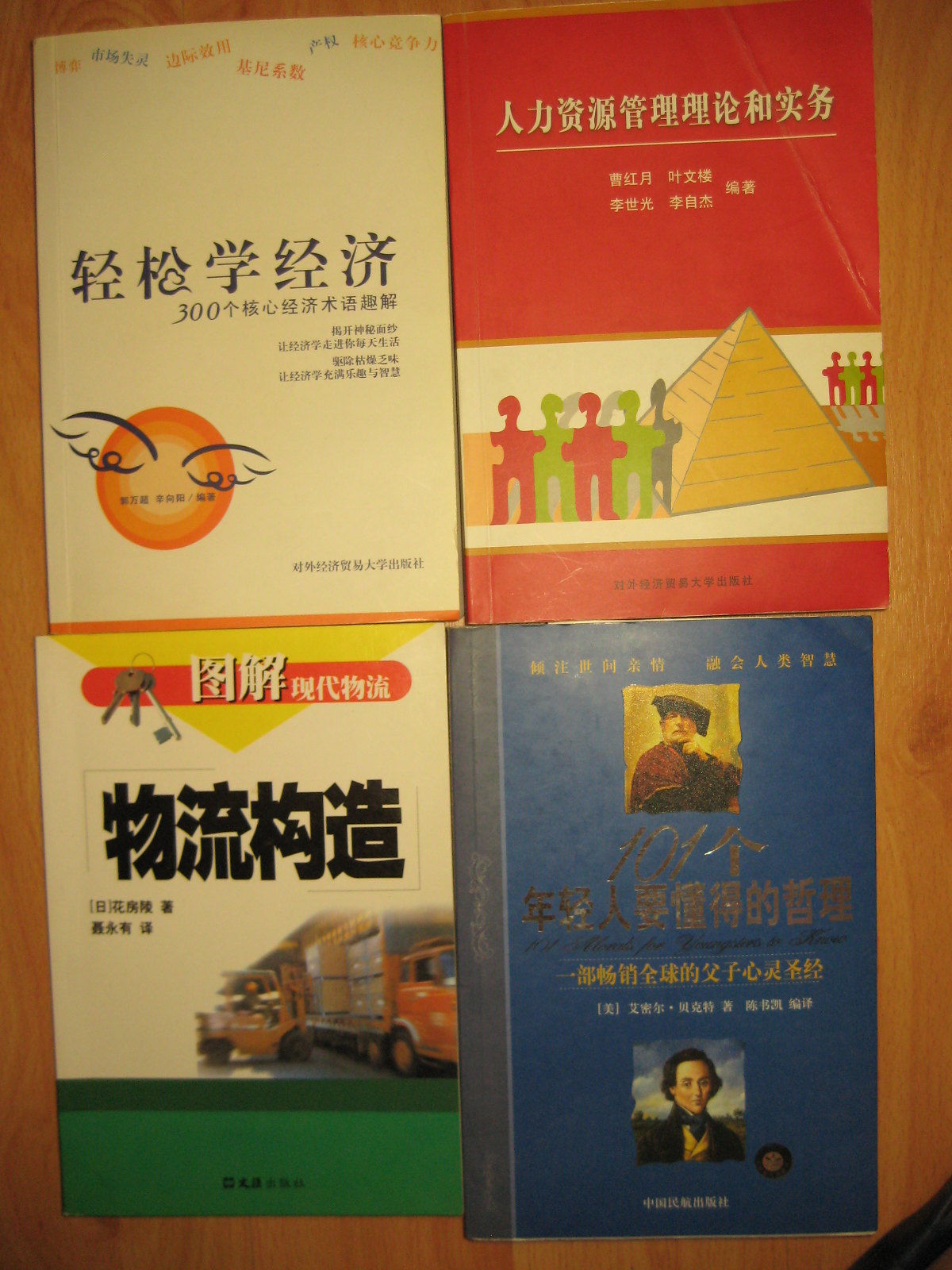This photograph features four well-worn books with aged bindings, written in what appears to be Japanese given the presence of kanji characters on their covers. The books' covers are diverse in both design and color: the top-left book is predominantly white with black text and an orange circle, giving little away about its subject matter. The top-right book stands out with its red cover and white font, featuring a pyramid and an array of figures or objects in red, green, and gray, possibly hinting at themes of sociology or social studies. The bottom-right book is solid blue and displays the portraits of two men in colonial-era clothing, suggesting it might be a history book. Lastly, the bottom-left book is multicolored with shades of white, green, red, and yellow, and depicts what resembles a forklift and boxes, suggesting it is likely a work manual or instructional guide. Though these books are old and their texts are unreadable to the observer, the imagery and design of their covers provide valuable hints about their possible contents.